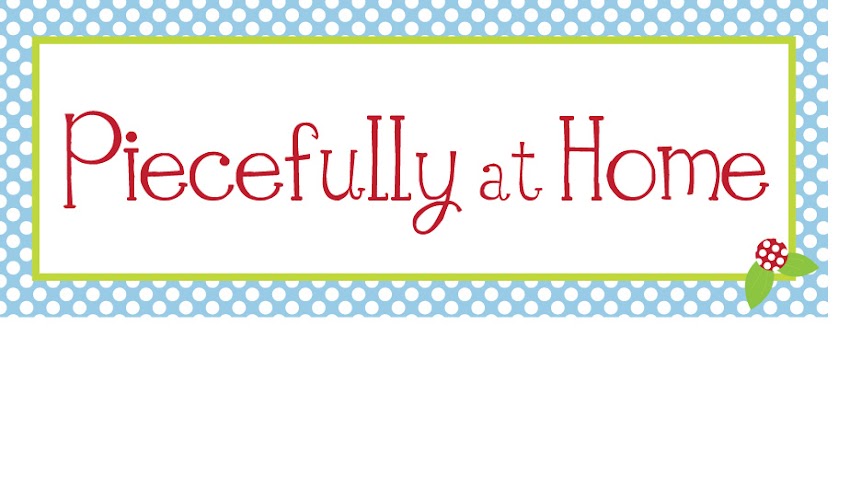The image is a digitally created banner with the phrase "Peacefully at Home" prominently displayed in the center in red lettering and a playful font. The banner features an intricate border, starting with a light blue edge decorated with white polka dots, reminiscent of small eggs. Inside this, there is a secondary lime green border that wraps around a white background where the text is located. At the bottom right corner, there's an illustration of a raspberry, depicted as a red circle with white polka dots and green leaves extending from each side, adding a charming detail to the composition. The overall design suggests it could be a decorative sign suitable for a classroom or home setting.